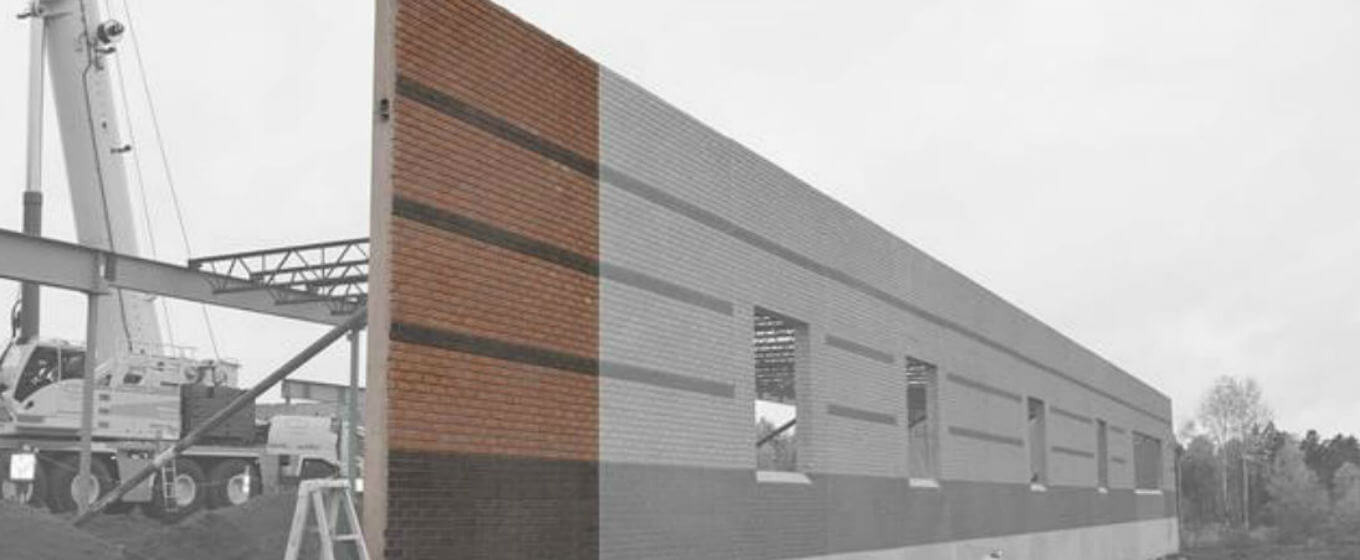The image captures a construction site, prominently featuring the front facade of an incomplete building with five windows. The facade is a mix of colors with the left side showcasing alternating red and black bricks, while the right side transitions into gray tones, giving it a partially black and white appearance. A striking line of darker bricks runs the length of the wall, with a thicker line at the base. The photo is taken in landscape orientation and shows significant construction activity, including big white cranes and steel supports that hold the facade upright. In the foreground to the left, a stepladder and some construction chucks are visible among the dug-up dirt, indicating ongoing groundwork. The sky above is white, creating a stark backdrop against the brickwork, while trees peep from the bottom right corner, adding a touch of nature to the scene.